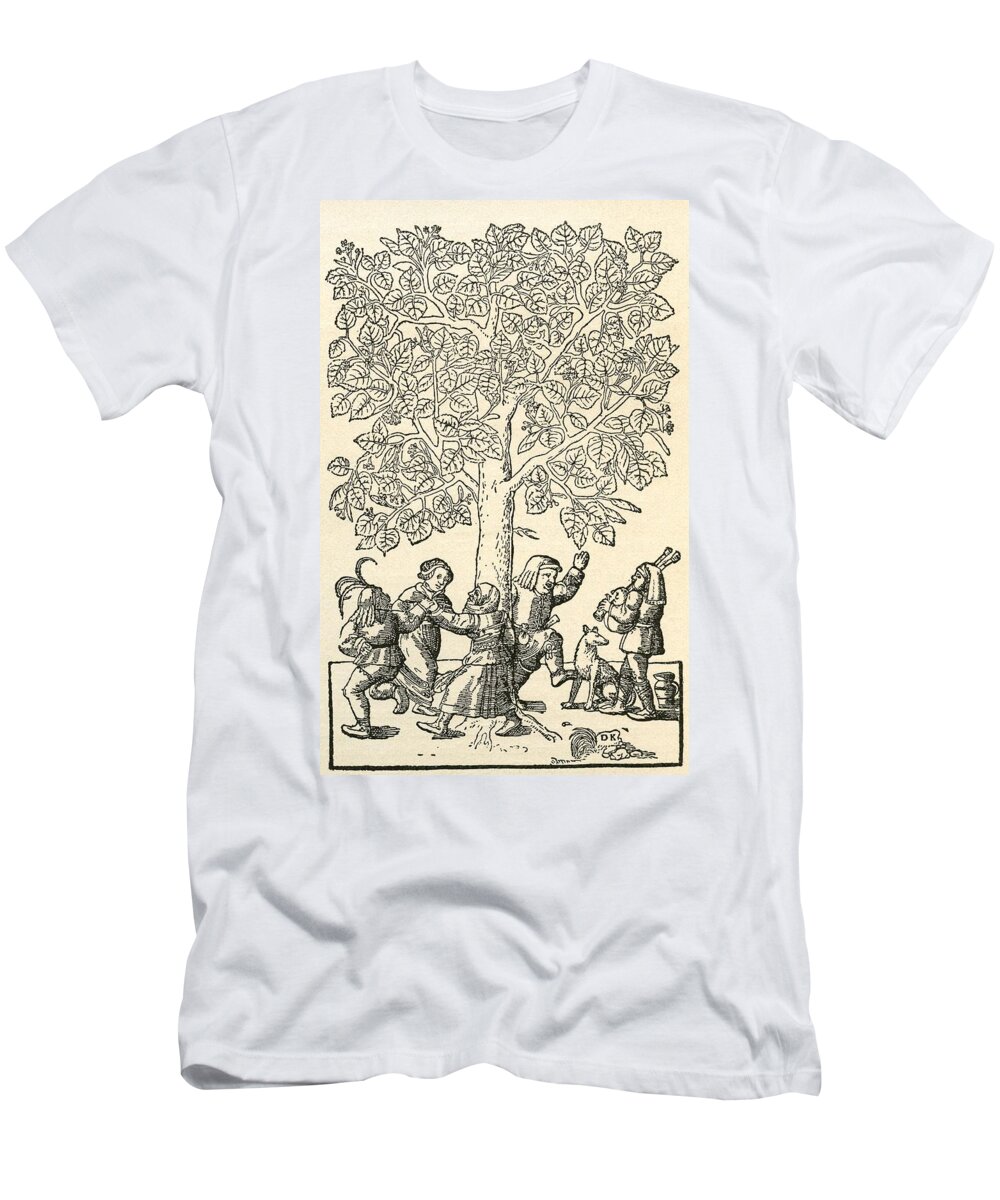The image depicts a staged, full-color photograph of a white, short-sleeve t-shirt laid out flat against a white background. The t-shirt is notably wrinkled, not neatly smoothed out. At the center of the t-shirt is a vertically rectangular artwork with a cream-colored background, featuring a detailed black ink sketch. The sketch illustrates a lively medieval scene with five people dancing around a tall tree with large leaves. The participants appear to be dressed in traditional attire, reminiscent of Pilgrims or people from the Middle Ages. Among the dancing figures, there's a man seemingly stomping the ground, and another individual on the right side playing bagpipes. A dog sits attentively below the bagpiper, gazing upward. On the far left, another person appears to be engaged in musical activity, contributing to the festive atmosphere of the scene.